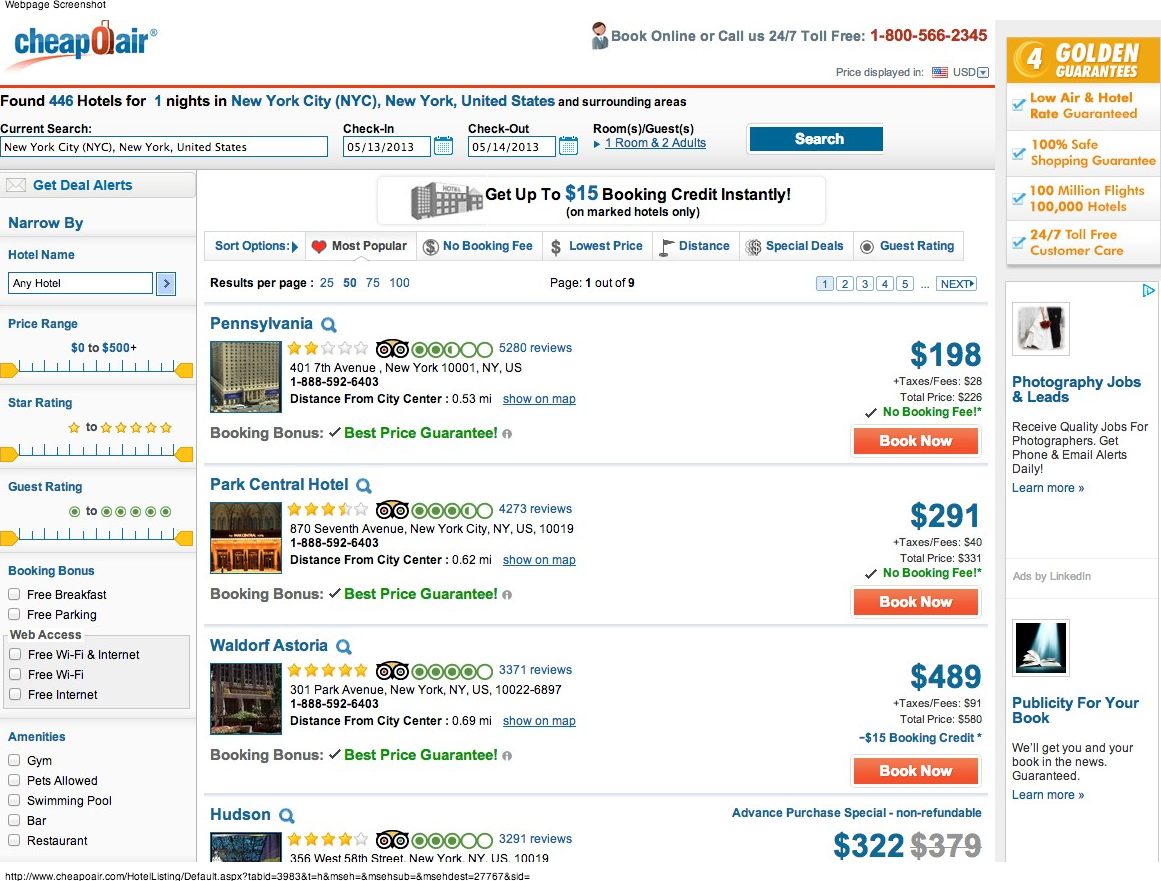This descriptive caption is for an image showcasing CheapOAir's hotel booking interface:

---

The screenshot displays the CheapOAir platform focused on hotel bookings. It features multiple categories such as "Most Popular," "No Booking Fee," "Lowest Price," "Distance," "Special Offers," and "Guest Rating." The hotels are listed with varying star ratings, starting from 2-star, ascending to 3-star, 4-star, and up to a 5-star hotel. One of the highlighted hotels is "The Hudson." 

Each hotel entry provides comprehensive details including its price range, star rating, and guest reviews. Additionally, visual representations like hotel images accompany each listing. Users have options to filter search results based on amenities such as free breakfast, free Wi-Fi, internet access, gym facilities, pet allowances, swimming pools, bars, and restaurants. 

The interface is laden with advertisements but retains functionality for searching specific dates, highlighting a check-in date of May 13, 2013, with the stay extending to the next day. Booking options are versatile, allowing for online reservations or phone bookings.